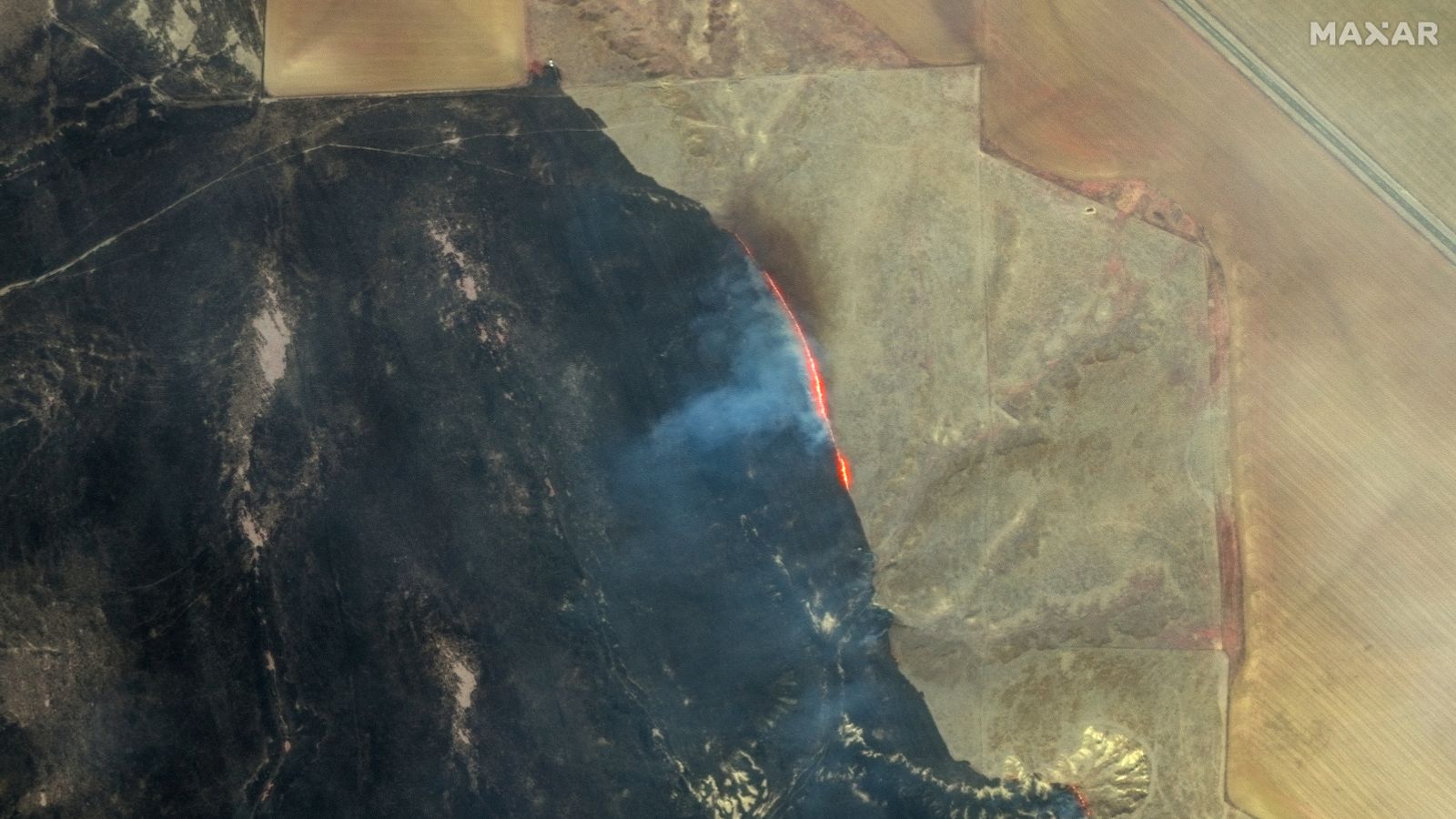This photo, taken from an aerial perspective, showcases a complex landscape that intertwines natural and human-made elements. The central focus is an area that appears rocky with various distinct color patterns and textures. To the right of the image, there is a light brown wood section giving way to a red quartz-like area. Adjacent to this is a strip of gray stone featuring a bright red line that transitions into a section of black granite, which has white accents scattered throughout. Toward the top right corner, there is a lighter brown material separated by a gray stripe, while on the top left corner, the black granite appears to have more pronounced white accents. There is also a medium-colored wood square located towards the top alignments of these elements.

Adding to the scene's complexity, the image has a dim, almost smoky quality, evoking a resemblance to a satellite photo of a forest fire, with dark, smoky ground areas, and fiery red sections suggesting active burning zones. Additionally, subtle details like striations resembling a farm field and possible water or past lava flows at the bottom enrich the scene. At the very top right corner, the word "Maxar" is visible, hinting that this might be a satellite image. 

The juxtaposition of light and dark areas, along with red lines and the perception of both rocky terrain and potential volcanic activity, suggests a dynamic and potentially hazardous landscape captured in a moment of intense natural activity.